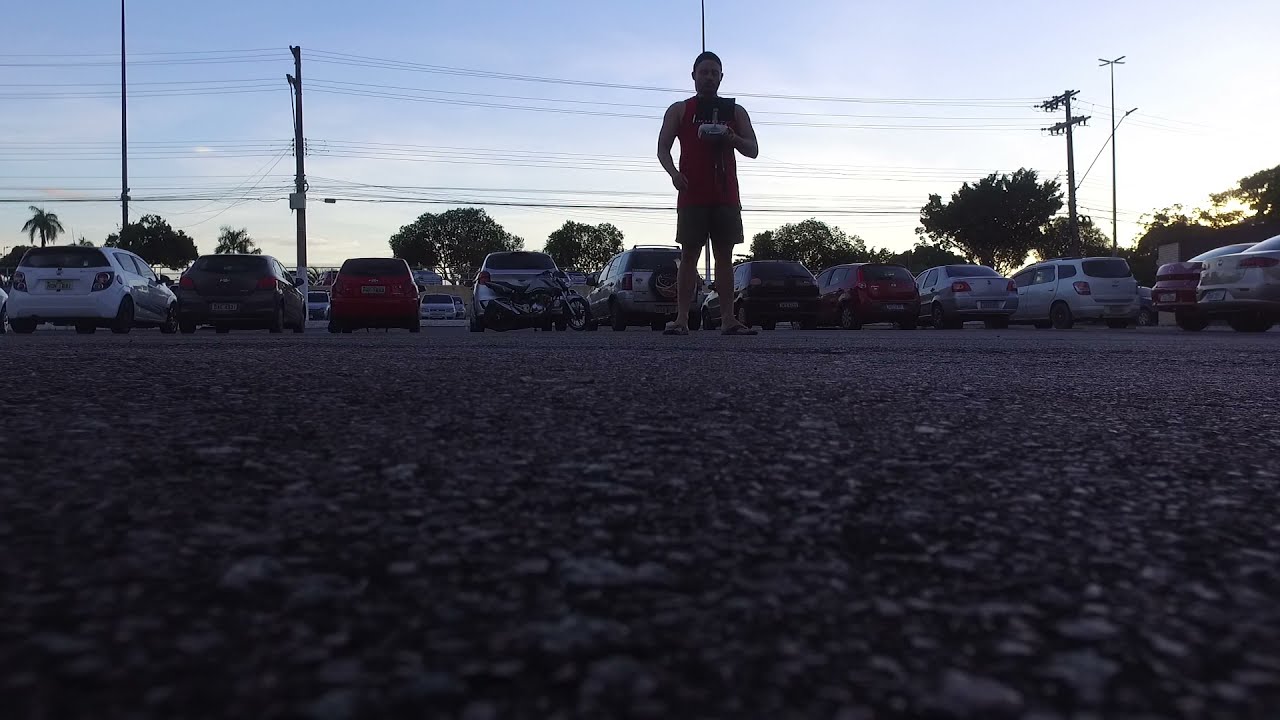The image is a color photograph in landscape orientation, capturing a scene in an asphalt parking lot during the twilight hours, either at dawn or dusk. The sky is a light blue, presenting a striking contrast against the silhouetted figure of a man standing centrally near the top of the frame. He is backlit by the low sun, which is either rising or setting behind a line of trees, creating a dramatic silhouette. The man, casually dressed in a red tank top, gray shorts, and sandals, appears to be holding a white controller, suggesting he might be operating an RC car or potentially a drone. The view is from a very low angle, as if the camera is placed on or near the ground, possibly attached to a small vehicle or drone. Numerous cars are parked in the background and to the sides, facing away from the viewer. Power lines traverse the sky horizontally, adding to the detailed realism of the scene. The overall composition, with its rich play of light and shadow, gives a sense of quiet anticipation, with the man and his device hinting at some pending action or event.